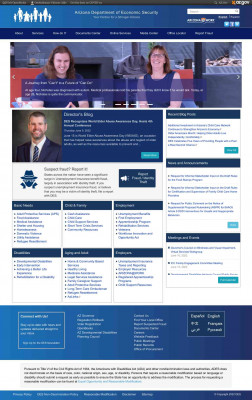Screenshot of an educational website captured on a mobile device, depicting a professional atmosphere. The main image at the forefront shows two women engaged in a joyous conversation – one in a blue shirt, the other in a sleeveless dress, standing in what seems like a modern building with glass windows. A computer is visible nearby. The woman in the blue shirt has her hands folded in a thoughtful posture, while the other woman's hands are not visible. Beneath this image is a brief article, though the text is too small to discern. Below the article, there is a photograph of a man dressed in a formal suit, complete with a white shirt, jacket, and tie, smiling warmly. The website itself features a color palette dominated by shades of blue – ranging from aqua to royal blue and dark blue. It's structured into various sections, each containing multiple links, making navigation comprehensive yet intricate. The site offers language options, being accessible in both English and Spanish. Despite the clarity of the design elements, the screenshot remains blurry, making details harder to distinguish.